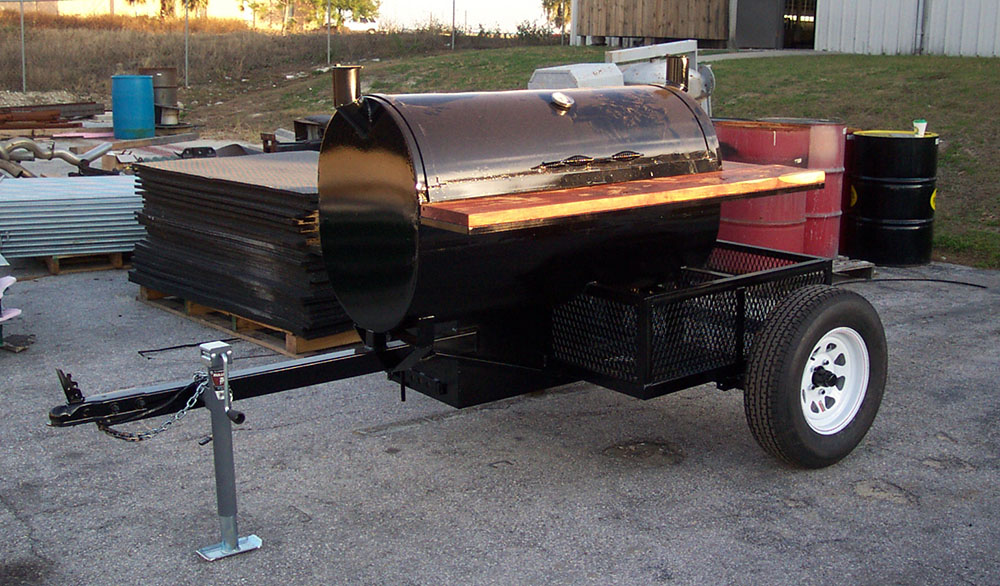The full-color outdoor photograph, taken during the day with natural light, features a horizontally rectangular image centered on a professional-grade portable grill mounted on a black trailer. This barrel smoker, characterized by its high-sheen cylindrical drum and equipped with a temperature gauge, is designed for easy transport, likely to barbecue competitions. The smoker, black in color, includes a wooden platform for cutting meat and organizing supplies and has smokestacks on either side. Surrounding the trailer are utility features like black wheels and a side basket for additional storage, as well as a latch and a trailer jack for vehicle attachment. The background consists of various outdoor elements, including some pallets, barrels possibly used for trash, scattered grass, a small hill, and a couple of trees in the upper left corner. Additionally, there's a modest wood building and shop area to the right, suggesting this site might be involved in manufacturing or storing these smokers.